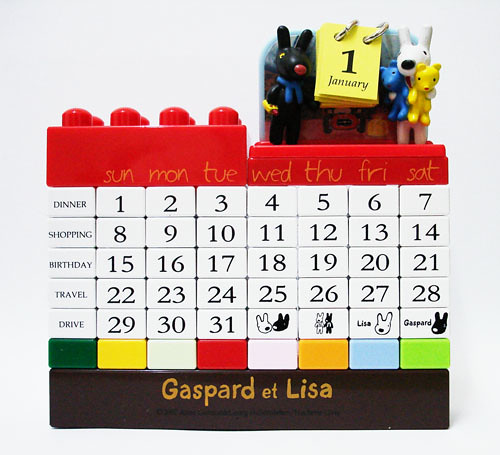This image portrays a creatively designed calendar reminiscent of Lego blocks, likely designed for or by children. Across the top of the calendar are two large red Lego blocks, each adorned with the days of the week, abbreviated in yellow as Sun, Mon, Tues, Wed, Thurs, Fri, and Sat. Flanking the left side of the calendar is a vertical column of white blocks labeled with various activities, including "Dinner," "Shopping," "Birthday," "Travel," and "Drive."

The core area of the calendar features numbered blocks representing the days of the month, starting with "1" and continuing sequentially along rows beneath each activity block. There are additional colored blocks in white, red, yellow, green, orange, and blue, adding a playful aesthetic.

Prominently, a yellow block situated next to the red Legos displays "January 1st," and the calendar is surrounded by charming cartoon characters: a white rabbit, a black rabbit, each holding yellow and blue teddy bears, respectively. At the bottom of the calendar, more detailed elements appear, including tiles with illustrations of two dogs, presumably named 'Lisa' and 'Gaspard,' correlating to the text "Gaspard et Lisa" printed at the base of the calendar.